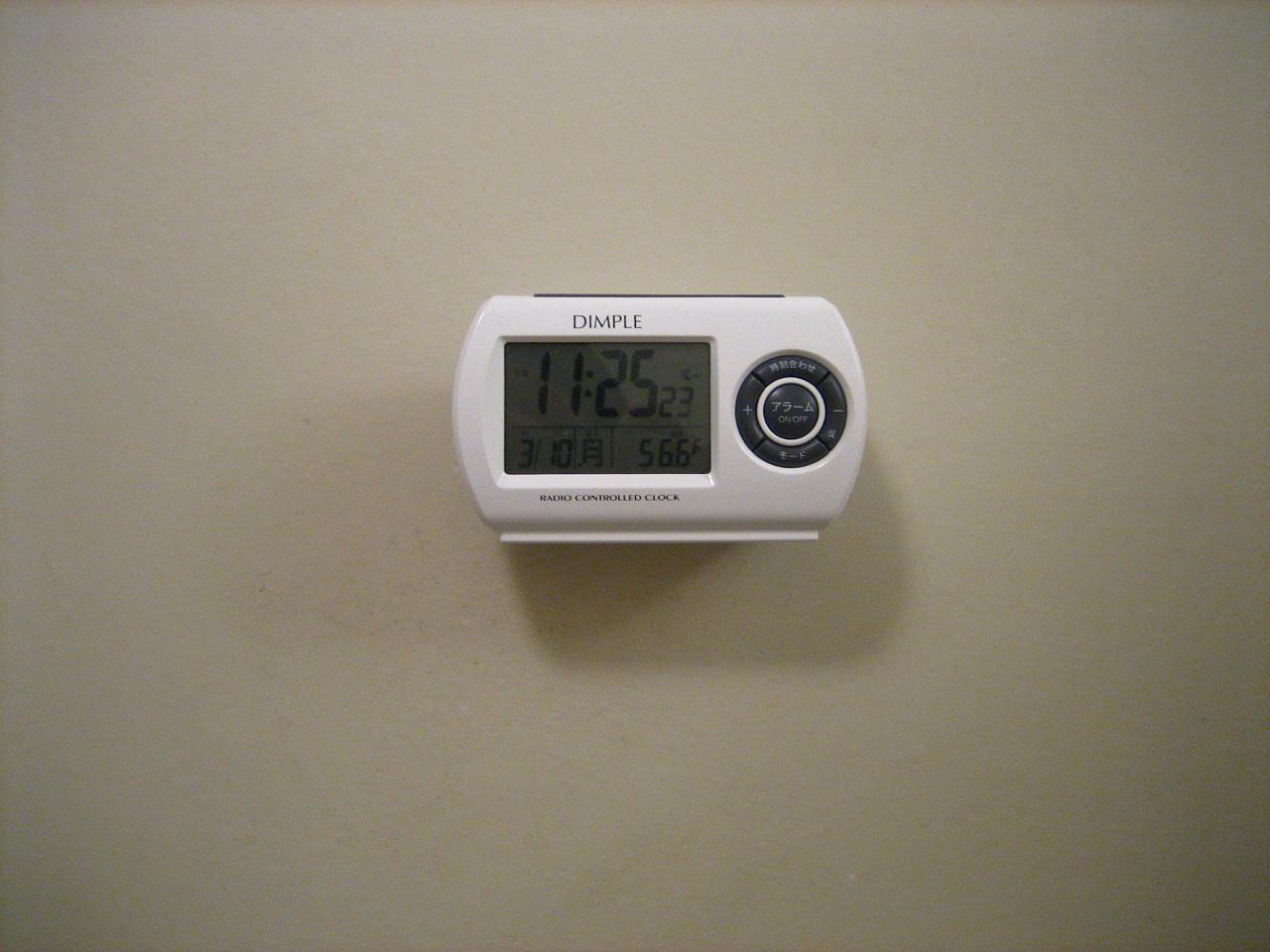The photograph features a sophisticated device mounted on a tan-colored wall. The wall's hue lightens at the center and subtly darkens towards the edges, incorporating hints of gray. The device, appearing to function both as a thermostat and a clock radio, possesses a unique design with rounded edges on its sides and straight lines at the top and bottom, giving it an almost oval-like shape.

Constructed of white plastic, the device prominently displays the word "DIMPLE" in black print at the top, indicating the brand, and "radio-controlled clock" at the bottom, describing its functionality. The digital screen, shaded gray, shows the time as "11:25:23" and the date "3/10" in the bottom corner. Additionally, the screen features a mysterious ladder-style icon and reads "56.6 F" at the bottom right, indicating the temperature in Fahrenheit.

Below the screen is a gray dial marked with a plus sign on the left and a minus sign on the right. Surrounding the dial, there are two gray buttons at the top and bottom, labeled in Japanese. A small white circle in the center houses another gray button inscribed with "on" and "off," accompanied by the corresponding Japanese characters.